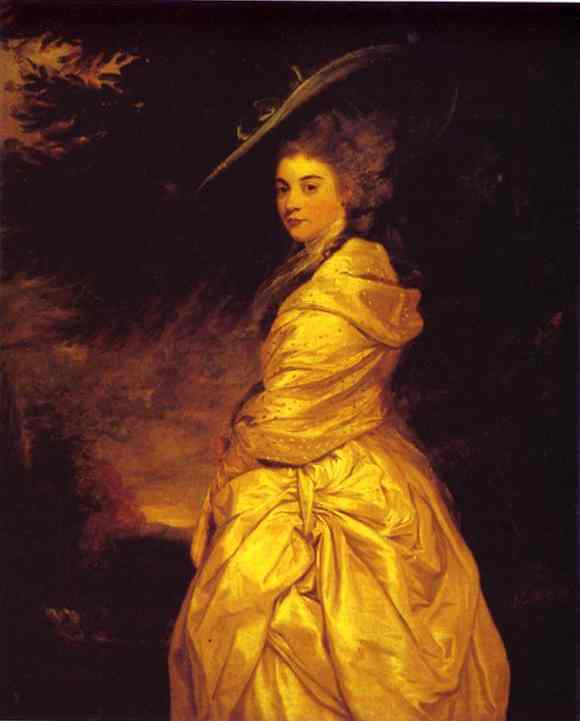This image is a detailed Renaissance painting of a young woman in her twenties with flowing brown hair cascading past her shoulders. She wears an ornate, golden wrap dress that drapes elegantly around her body in several sumptuous layers. Atop her head sits a wide-brimmed hat, tilted slightly downwards, adding to her air of sophistication.

The woman stands amidst a dark, textured backdrop featuring a blend of trees, branches, and subtle floral elements, which enhance the painting's intricate depth. Small openings in the backdrop suggest a glimpse of sky. The overall color palette is a harmonious mixture of browns, golds, and blacks, rendering the scene almost monochrome, yet richly detailed.

The young woman, captured mid-step, glances over her left shoulder with a curious expression, her head slightly tilted as if something has caught her eye. This pose subtly nods to the themes of class and elegance, characteristic of paintings depicting nobility. Her gaze not only adds a dynamic quality to the portrait but also engages the viewer, drawing them into the historical ambiance of the piece.